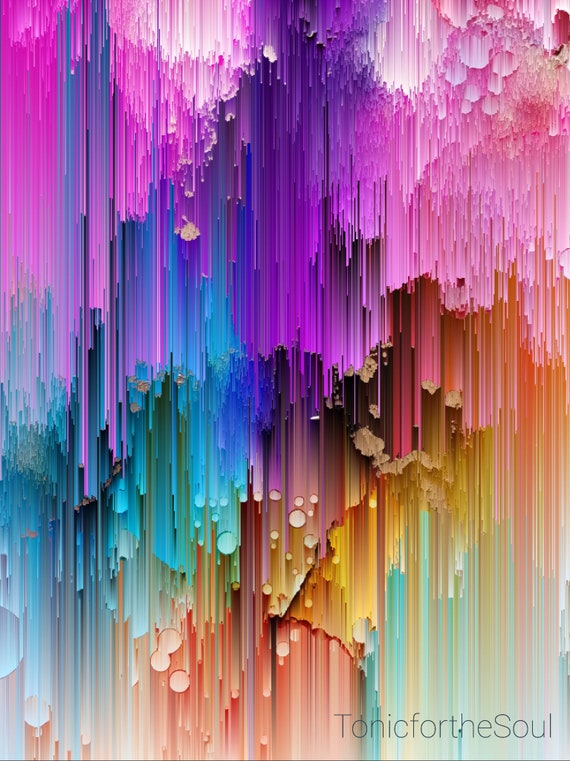This is an artistic illustration featuring an array of vibrant, straw-shaped lines that resemble dripping paint in a rainbow of colors, descending from the top of the image. The colors are organized in sections that blend together subtly but are distinguishable by their hues, including various shades of pink, purple, red, orange, yellow, blue, and teal. Towards the bottom of the image, the colors become lighter and more subdued. Interspersed with the colorful lines are whitish beige, bubbly shapes that appear to float in front of the lines, adding depth and dimension. The bottom right corner of the illustration features the overlay text “tonic for the soul.” The entire composition is very vibrant and unique, blending elements of both painting and illustration in a captivating visual display.